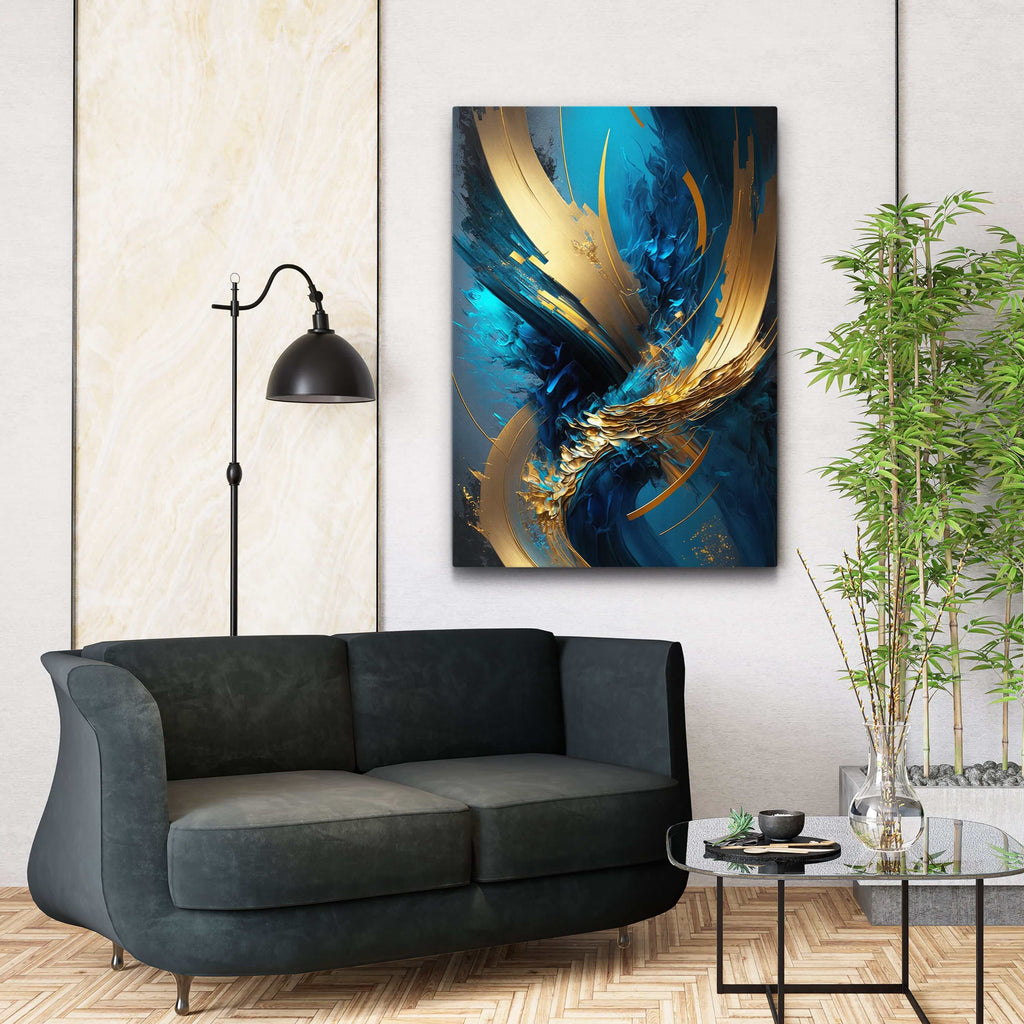This image depicts a modern and well-decorated living room. The focal point is a dark gray fabric loveseat, comfortably placed against a wall adorned with a striking abstract painting. The painting stands vertically and features splashes of metallic blue and gold, resembling an explosion of paint. The loveseat is complemented by a sleek black floor lamp with a downward-hanging black lampshade to the left.

On the floor, a light wood-patterned tile with a zigzagging design, possibly bamboo, adds a touch of contemporary style. In front of the loveseat sits a small, square glass coffee table featuring a clear glass vase with bamboo shoots and thin green leaves. Additionally, a cup of tea rests on a wooden coaster. 

To the right of the loveseat, a gray stone planter containing gray stones supports more bamboo shoots, enhancing the serene ambiance of the space. The overall setting suggests a modern, minimalistic home environment.